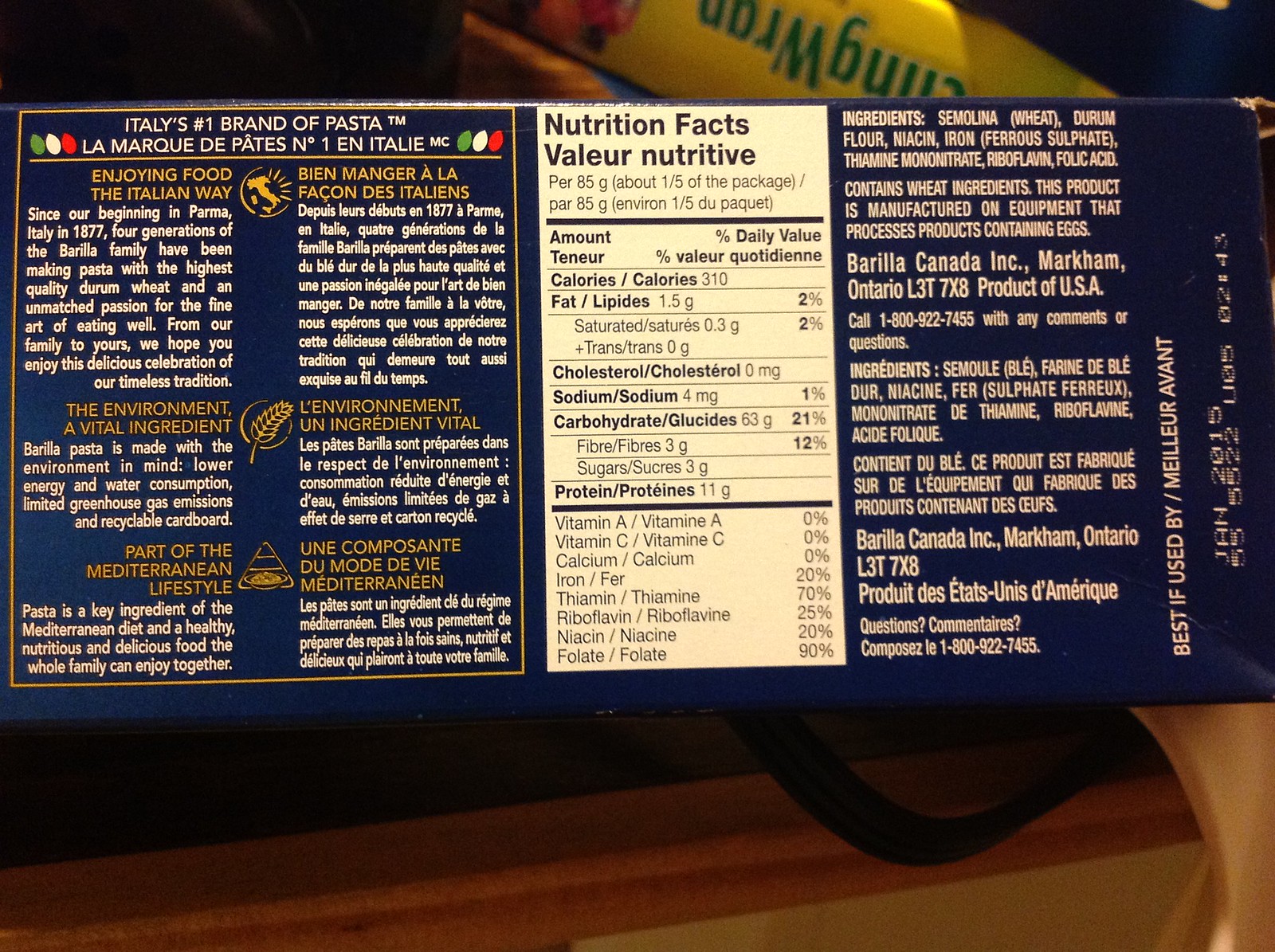Caption: 

A close-up of a pasta product label, presented in a striking blue background adorned with white text and brown descriptors. The left side of the label features bilingual content, possibly including English and Italian, or even French. At the top, a prominent declaration states, "Italy's Number 1 Brand of Pasta," clearly indicating the product's high standing. The central section of the label displays the nutrition facts within a standard white rectangular box, providing detailed percentages and daily values. The right side outlines the ingredients in white text, specifying the product's origin from Markham, Ontario, yet noting it as a product of the USA. Additionally, the best by date is clearly marked on the right side, indicating the product should be consumed by January 2015.